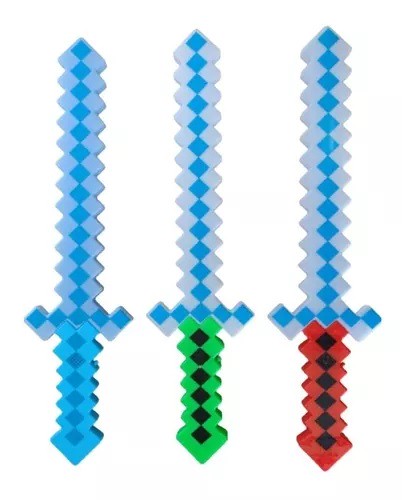The image showcases three digital, pixelated long swords, reminiscent of those found in Minecraft-style games. Arranged vertically with their handles at the bottom and tips pointing upwards, each sword is crafted from square-shaped or diamond-shaped pixels, giving them a serrated knife appearance. The left sword features a vibrant turquoise blue handle, transitioning to a mix of light and dark blue squares forming the blade. The middle sword displays a handle made of black and green squares, leading up to a blade composed of alternating white and blue squares. The right sword sports a red and black handle, with a blade similar to the middle sword, featuring blue squares along its length. All three swords are set against a plain white background, emphasizing their pixelated, geometric design. The entire image has a clear but intentionally pixelated digital art style, common in gaming visuals.